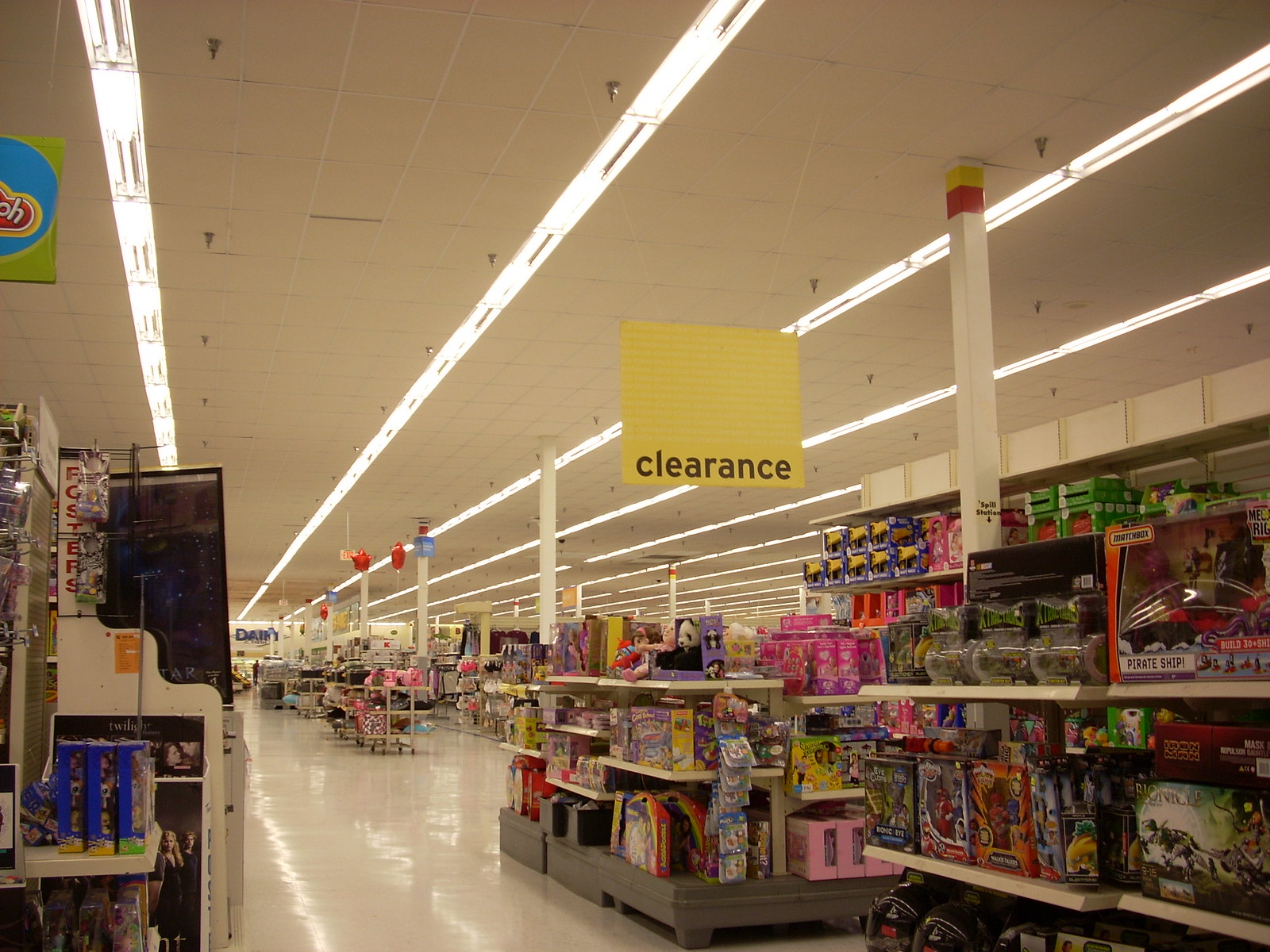The image depicts the interior of a store, capturing a well-lit aisle section. On the right side of the aisle, there are shelves stocked with various toys, adding a vibrant and colorful aspect to the scene. Further down the aisle, there's a central section displaying a prominent yellow sign hanging from the ceiling that reads "Clearance." The capture includes both the floor and ceiling, providing a comprehensive view of the store's layout. Additional middle aisle sections are visible further down the corridor. To the left, the edge of another aisle can be seen, giving a sense of the store's extensive and organized arrangement.